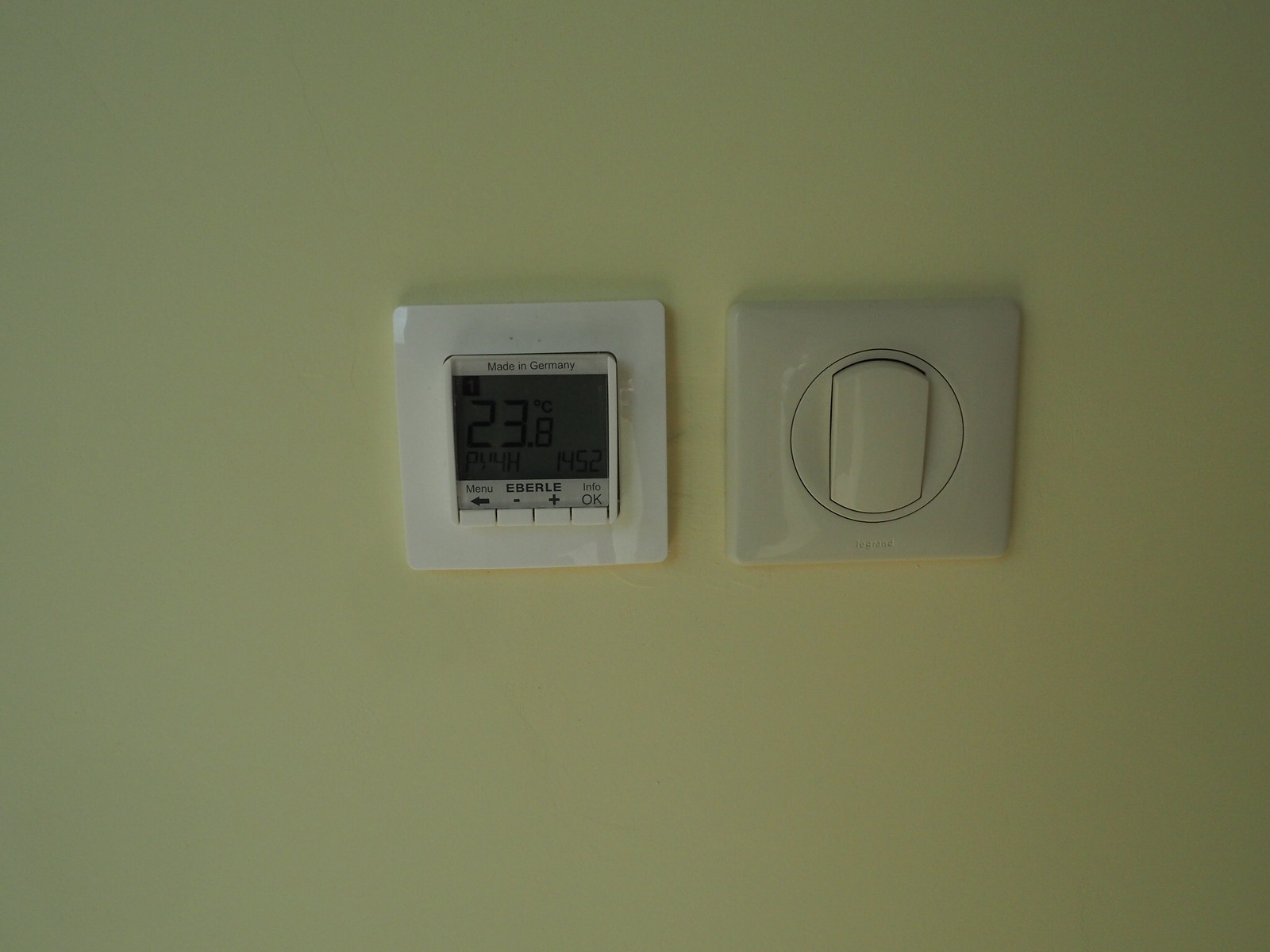This image showcases a background wall in a yellowish-beige shade, accentuated by subtle variations in lighting and shadows. The surface appears relatively smooth, though it may possess some minor texture typical of walls, which isn't prominently visible.

Centrally located on the wall is a small, white, rectangular panel with a cut-out section in the middle. This panel displays multiple elements: at the top, a gray strip bears the text "Made in Germany." Below it is a digital display resembling an alarm clock screen, indicating the number "23.8" in black along with additional smaller black numbers beneath it. 

Further down the panel, another gray strip presents several button functions labeled "Menu," "Everly," "Info," and more. Adjacent to these labels are four small white buttons, adding to the panel's functionality.

To the side of this panel, there is an old-fashioned light switch in a tan beige hue, featuring rounded edges and a circular center with a protruding switch that can be toggled up or down. This contrast in design elements creates an interesting visual dynamic on the otherwise neutral background wall.